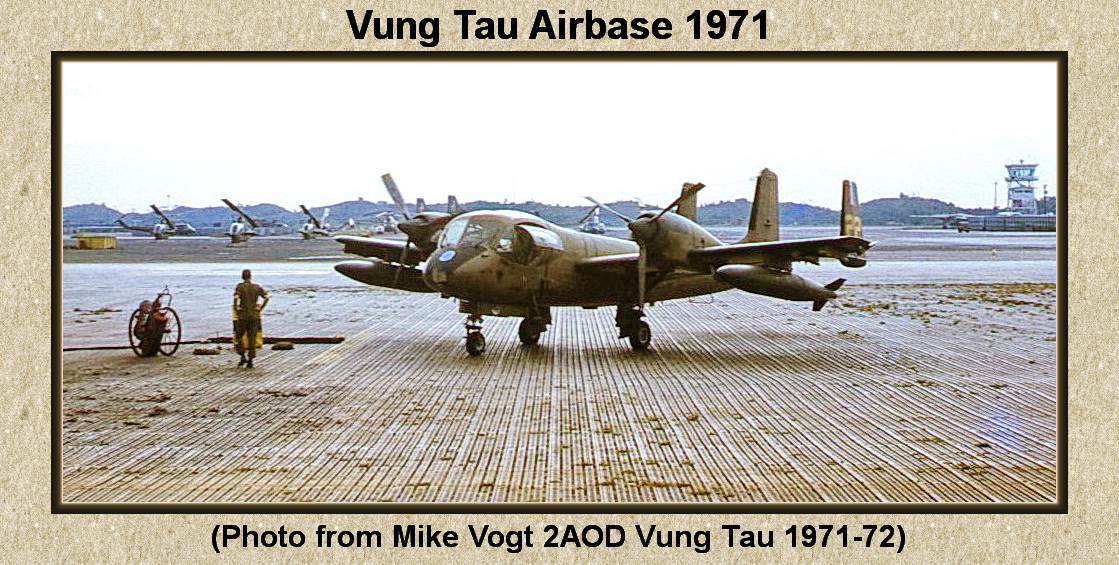This outdoor daytime photograph captures a detailed scene at Vung Tau Air Base in 1971. In the foreground, a stationary olive green military aircraft, equipped with two propellers and rockets or bombs on each wing, rests on a grid-patterned runway. A man in an olive green military uniform stands to the left of the aircraft, with his back to the camera and hands on his hips. Beside him, a large tank mounted on wheels is visible. In the background, there are additional small aircraft and helicopters along with a scenic view of a mountain range and a harbor featuring a series of mounted cannons. The distant landscape includes a watchtower and is set against a gray sky. This photograph, bordered in beige, has captions on the top and bottom: "Vung Tau Air Base, 1971" and "Photo by Mike Vogt, 2 AOD, Vung Tau, 1971-72."